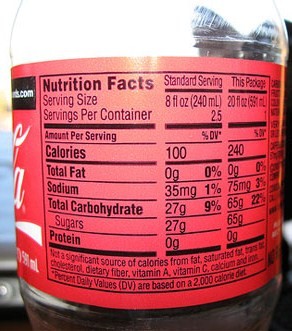This image features a clear, empty 20-ounce Coca-Cola bottle made of plastic. The prominent red label partially displays the iconic Coca-Cola logo, with visible letters 'L' and 'A' accompanied by a white stripe beneath them. The back of the red label reveals detailed nutritional information printed in black. It indicates that the serving size is 8 fluid ounces, with approximately 2.5 servings per container, and a total volume of 20 fluid ounces. The label details the caloric content as 100 calories per serving, totaling 240 calories per container. It mentions that there is no fat content. The sodium content is specified as 35 mg per serving and 75 mg per container. The total carbohydrates and sugars are both listed as 27 grams per serving, amounting to 65 grams per container, with no protein listed.